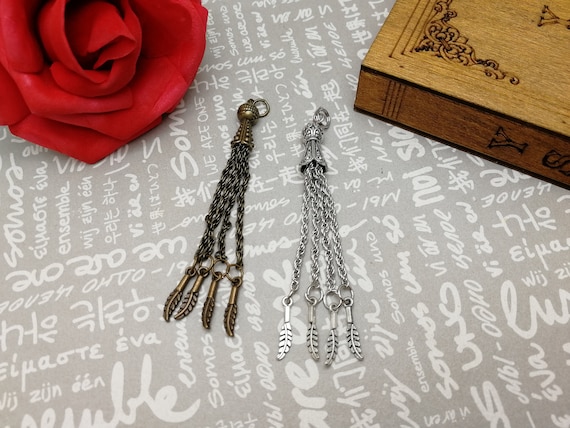This detailed photograph showcases two long, dangly earrings of identical design but distinct materials. The earring on the left flaunts a rich bronze hue, while the one on the right gleams in silver. Each earring features a central pendant from which four delicate chains dangle, each concluding with a petite, intricately fashioned metal leaf pendant. The background is a medium-light gray fabric adorned with white text in various languages, contributing an international flair. In the upper left corner, a fully-bloomed red rose adds a touch of natural beauty, contrasting with the upper right corner where a medium-color wooden box, possibly a jewelry or cigar box, provides a rustic charm. The box appears to have some design work etched into it, including partial letters “Y” and “S.”